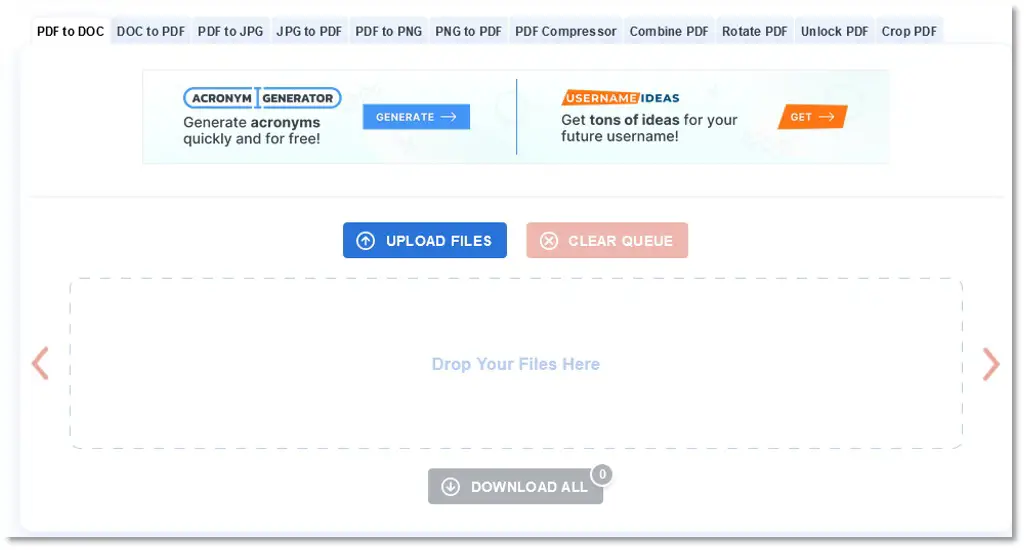Screenshot of a versatile data converter application interface. At the top of the interface, users can select from various conversion options including PDF to DOC, DOC to PDF, PDF to JPEG, JPEG to PDF, PDF to PNG, and PNG to PDF, among others. The main section of the screen is dedicated to uploading files, which can be done either by clicking the prominent blue 'Upload' button or by dragging and dropping files into the designated middle area. Once files are uploaded and converted, they can be collectively downloaded by clicking the gray 'Download All' button, located just beneath the main upload area. The interface is user-friendly and efficiently designed for seamless file conversion.